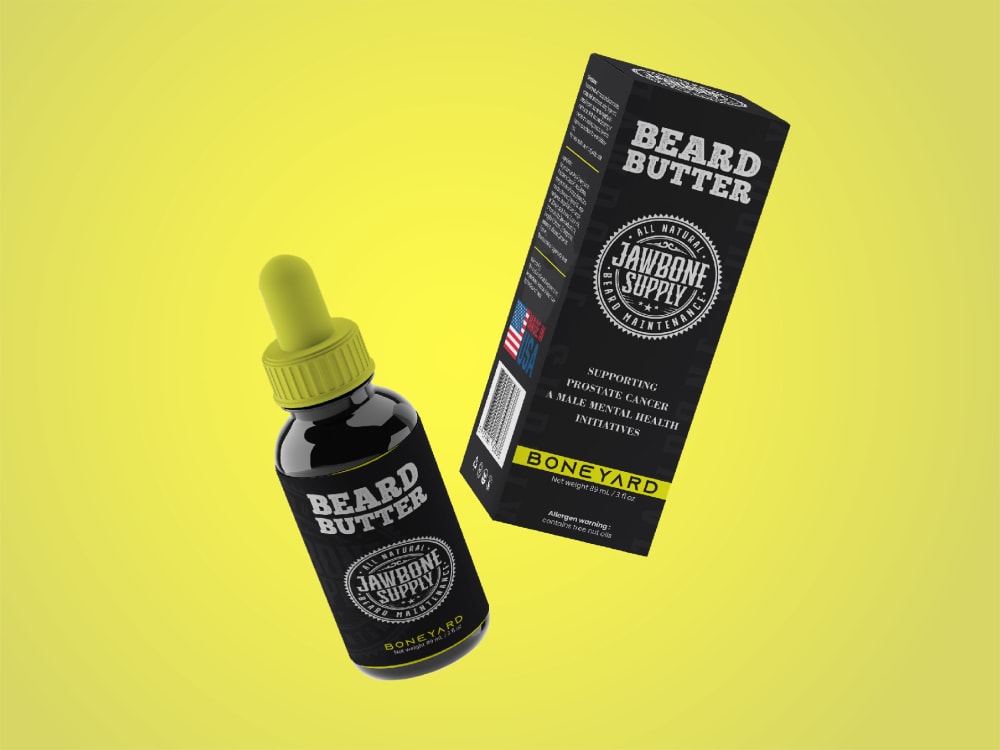The image features a carefully arranged display of a product consisting of a cylinder-shaped black dropper bottle and its corresponding retail box. The bottle is tilted slightly to the left, with the top pointing toward the upper-left corner of the image. The cap of the bottle, which is a bright yellow color, is designed to be unscrewed, revealing an attached dropper for dispensing the liquid. The dropper top, also yellow, can be squeezed to release the contents. Positioned to the right of the bottle is the product's box, designed with branding that reads "Jawbone Supply Beard Butter." Both the box and the bottle have this brand name prominently displayed, indicating the product is intended for beard care.